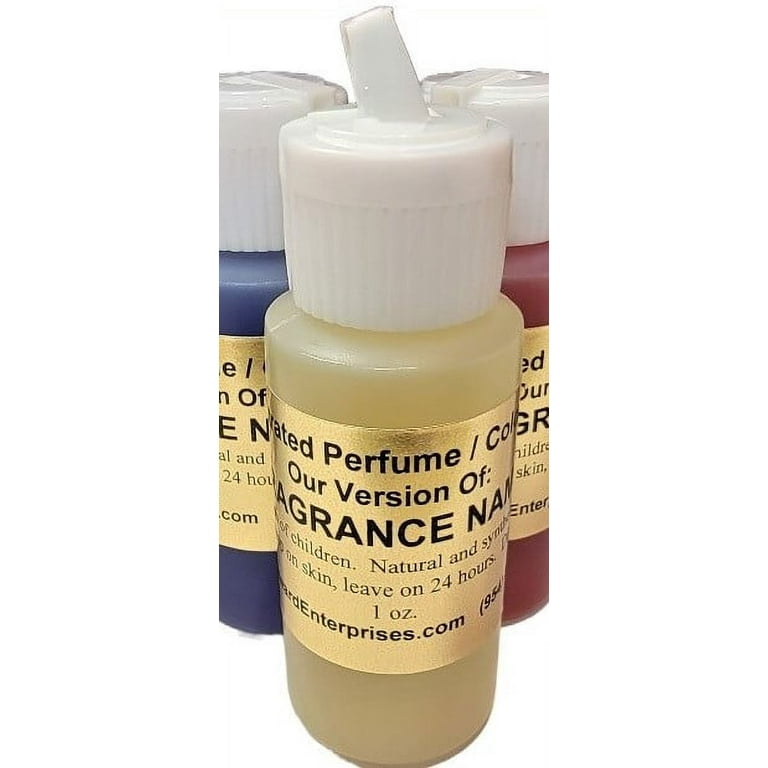The image features three small plastic bottles arranged in a triangle on a white background. Each bottle has a white screw cap with a pull-up nozzle, and they contain liquids of different colors: the bottle in front and center holds a tan liquid, the one on the left has a dark blue liquid, and the one on the right contains a red liquid. All bottles are clear plastic cylinders approximately two to three inches tall, adorned with a gold label featuring black text. The visible text on the label of the bottle in the middle reads at the top "Perfume," followed by "Our version of Fragrance," and then "Children, natural." Further down, it states "Leave on 24 hours," and "One ounce," with the last line partially revealing a website address.